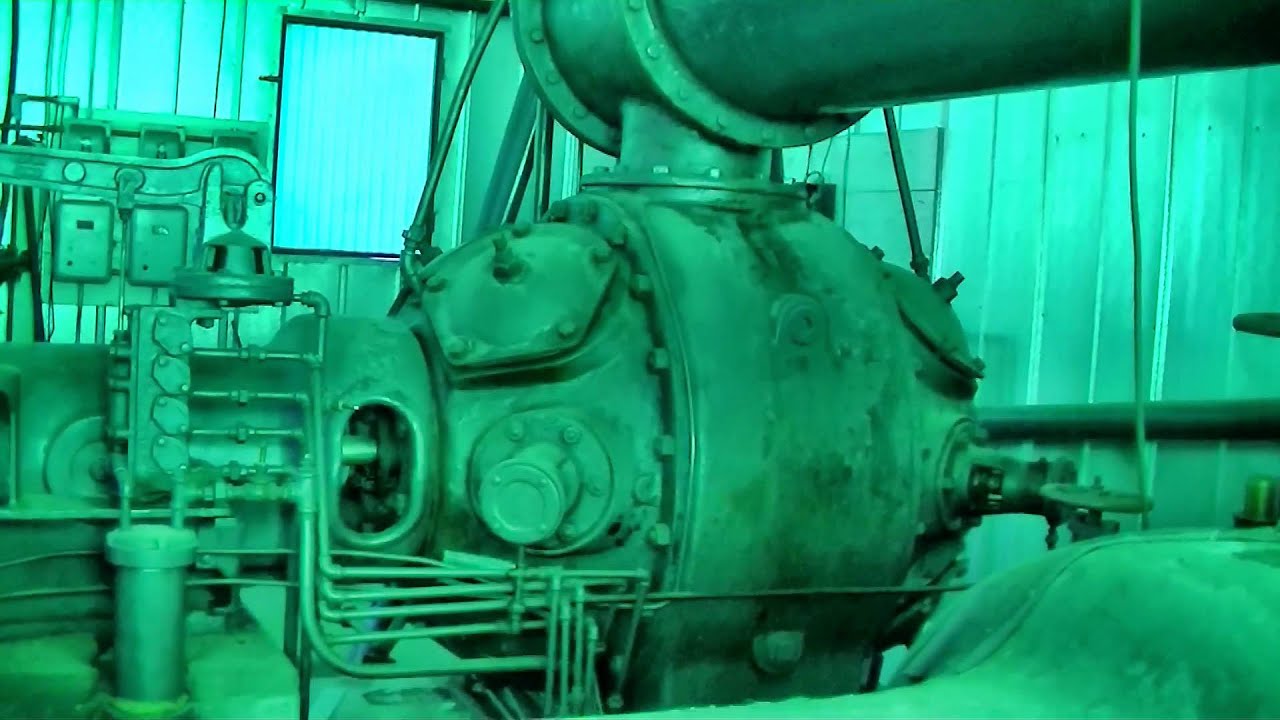An expansive, industrial pump station dominates the scene with its intricate network of pipes and robust machinery, all covered in a distinct blue-green hue. The centerpiece is a massive, green-tinted engine, likely used for pumping operations, flanked by numerous tubes and conduits extending in various directions. At the apex of this colossal engine, an orifice connects to an additional pipe, suggesting a complex fluid transmission system, perhaps typical of environments such as a boiler room or a maritime vessel. In the background, to the left, a window reveals a glimpse of the clear blue sky, contrasting sharply with the overall monochromatic, bluish-green tint of the machinery.